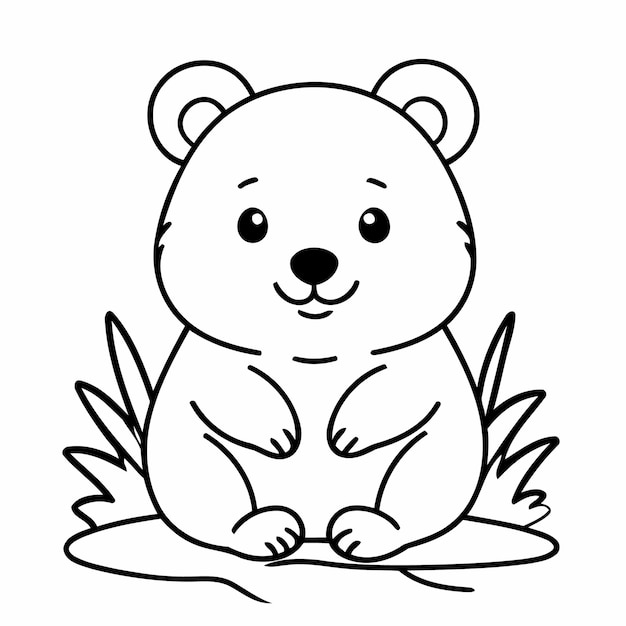The image is a black and white cartoon illustration of a small bear, reminiscent of a children's coloring book page. The simplistic design features a bear with a round, cutesy face adorned with two round, beady eyes that have small white dots for pupils, giving it a lively look. It has small, semicircular ears on either side of its head, and a brownish nose with simple lines indicating nostrils. Its mouth, formed by a small half-circle, adds to its adorably innocent expression. The bear is depicted sitting on its butt with its arms and feet tucked in front of it, creating a circular, cuddly appearance. Grass or oval-shaped lines sprout around its sides and it appears to be sitting on a platform or lily pad. The entire drawing is composed of clear black outlines against a plain white background, making it perfect for a child's coloring activity.